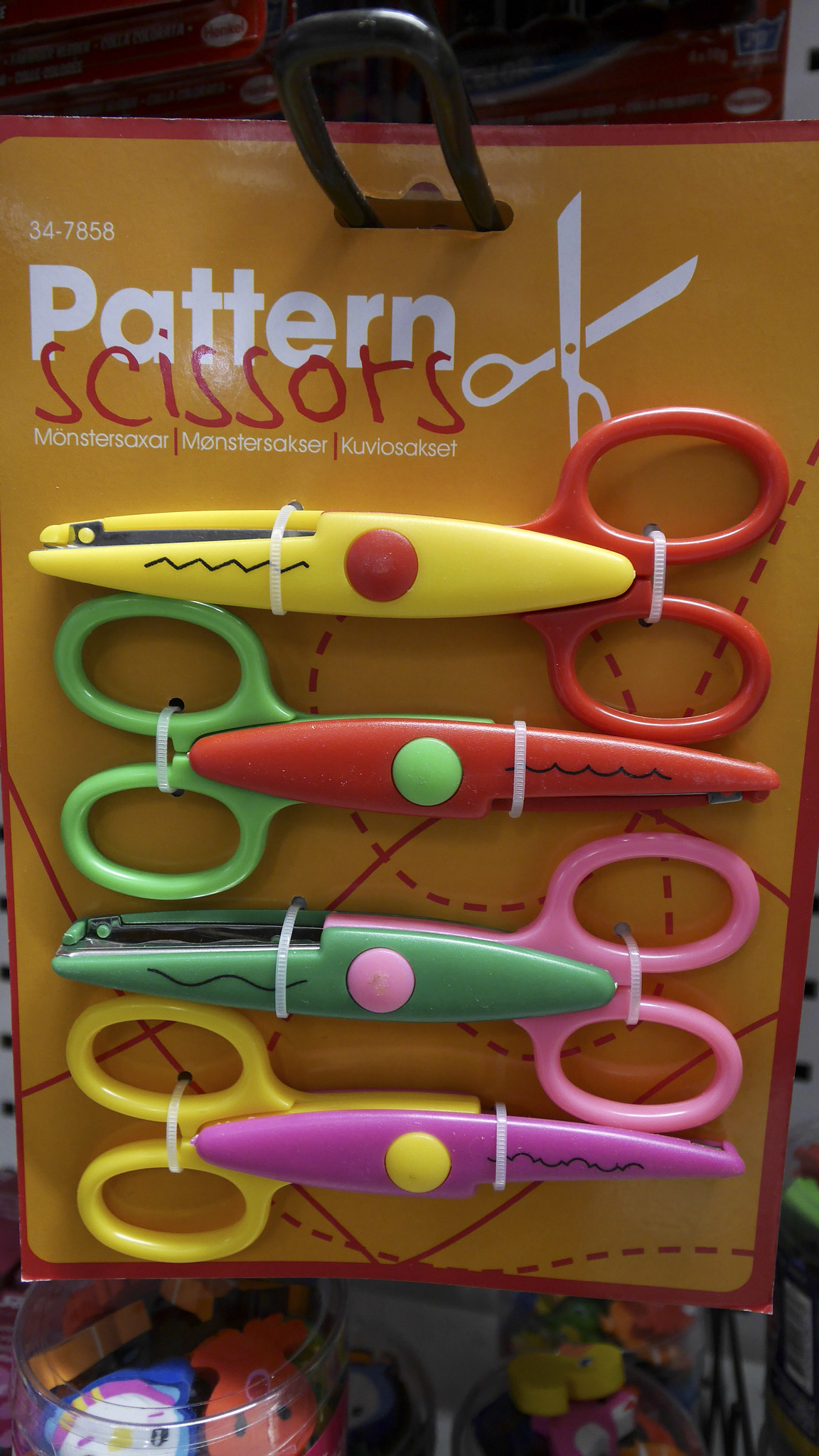In this image, we see a package of four colorful pattern scissors displayed for sale in a store. The scissors are zip-tied to a cardboard backing with white zip ties, which keep them securely fastened without any plastic covering. Each pair features distinct color combinations and the handles alternate direction with each scissor. The top pair has yellow blades with a red handle, followed by red blades with a green handle, then green blades with a pink handle, and finally pink blades with a yellow handle. The packaging clearly reads "34-7858 Pattern Scissors," with "Pattern" written in white and "Scissors" in red. There's also a logo depicting a pair of scissors pointing to the upper right-hand corner of the packaging. Additional miscellaneous items, potentially in jars or jugs, can be seen at the bottom of the image, also for sale.